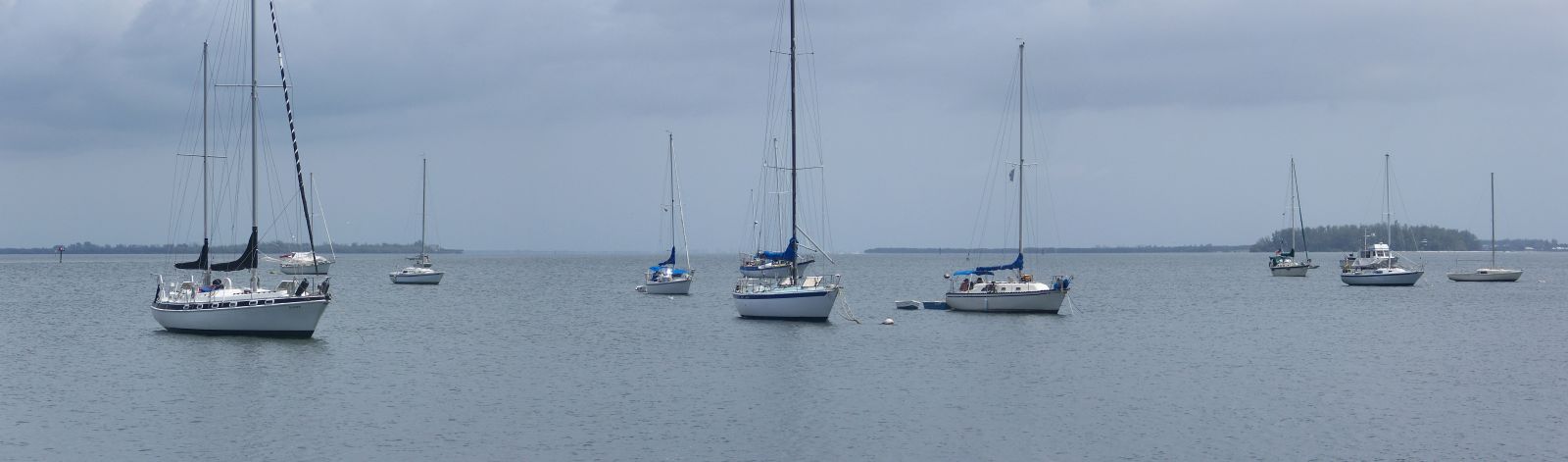This panoramic image features a serene seascape dominated by about 11 sailboats peacefully floating on a calm, bluish-gray waterway. The sailboats, all white with their sails retracted, are arranged in clusters throughout the scene, some closer in the foreground and others appearing smaller in the distance. The water exhibits slight ripples but no significant waves, enhancing the overall tranquil feeling. 

The sky is overcast with heavy, low-hanging clouds that possess a grayish-blue hue, mirroring the color of the water below. In the distant background, several islands or peninsulas covered with green foliage are faintly visible, adding depth to the horizon. Despite the lack of vivid colors and the gray, somber atmosphere, the image captures a subtle beauty in its stillness and the harmony of the anchored boats waiting together on the quiet waters. There is no text or signing on the photo, allowing the viewer to fully immerse in this calm and contemplative maritime scene.